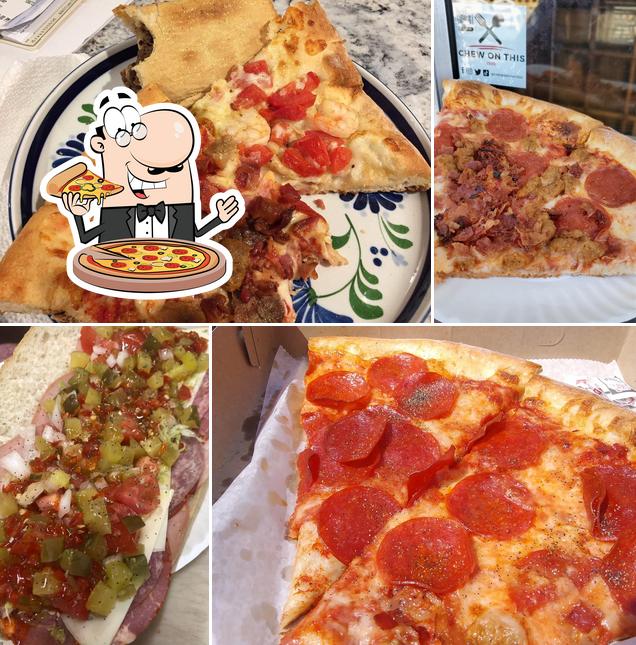A composite advertisement for a pizza shop, arranged in a square format with four distinct images. The larger images are placed at the top left and bottom right, while the smaller ones occupy the bottom left and top right.

- **Top Left Image**: A delectable pizza displayed on a decorative glass plate, partially obscured by a whimsical cartoon character in the bottom left corner. The character, with exaggerated features like a huge nose, glasses, and a mustache, is dressed in a black suit and bowtie. He exudes joy as he holds a slice of pizza, emphasizing the enjoyment of the meal.

- **Bottom Left Image**: A mouthwatering sandwich brimming with colorful, chopped vegetables, adding a fresh and vibrant touch to the assortment.

- **Bottom Right Image**: Two appetizing slices of pepperoni pizza laid out on white wax parchment paper, showcasing the classic flavor combination.

- **Top Right Image**: Another set of pizza slices, topped with pepperoni and additional ingredients, displayed on a convenient paper plate.

Together, these images create a visually engaging and enticing display that highlights the variety and quality of options available at the pizza shop.